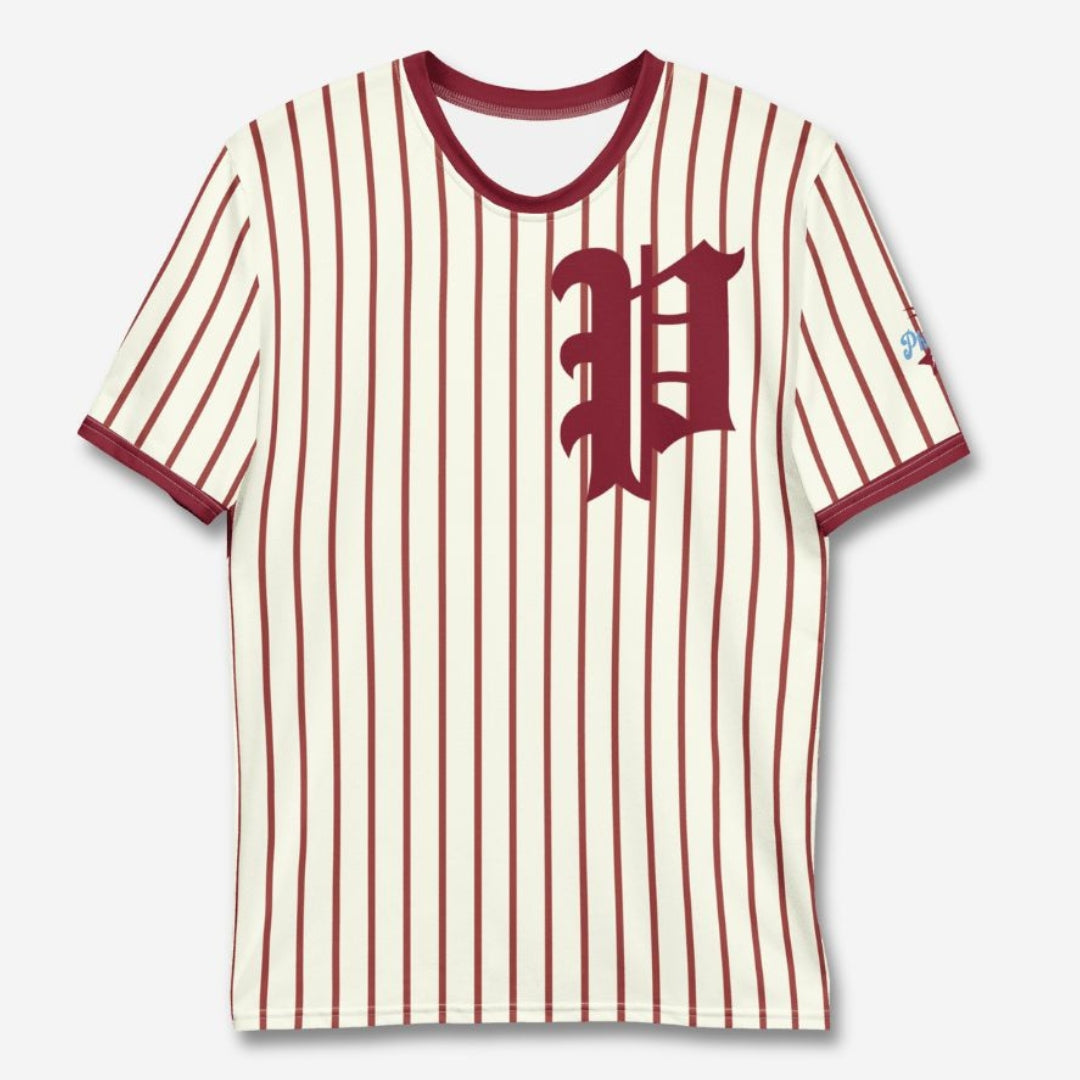This photograph features a vintage-style Philadelphia Phillies baseball jersey displayed on a white background. The jersey is predominantly white with thin, vertical red stripes. It has short sleeves accented with deep burgundy red trim around the cuffs and a matching reinforced collar. Prominently displayed on the left chest is a large stylized "P," rendered in an old English font, measuring approximately six to seven inches in both length and width. The left short sleeve also features a small blue patch with indistinct writing, likely related to the team. The jersey captures a classic design with emphasis on the fine red stripes and distinctive "P," indicative of the Philadelphia Phillies.